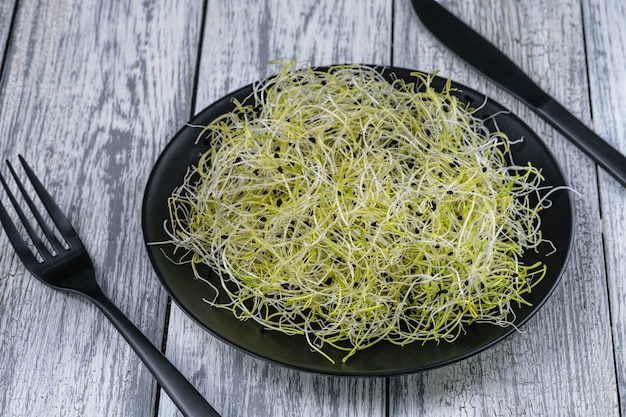A black, round plate sits on a wooden table made of white and gray panels. On the plate, a heap of white and yellow sprouts, potentially alfalfa, are interspersed with tiny black sesame seeds. The sprouts are characterized by their long, filament-like strands, with lighter green tips and translucent white bases. To the right of the plate lies a black knife, paralleled by a black fork on the left side, both pieces of black cutlery seemingly from the same set. The table beneath the plate resembles a picnic table with its distinct wood grain pattern, offering a rustic yet appealing backdrop to this minimalist, vegetarian dish.